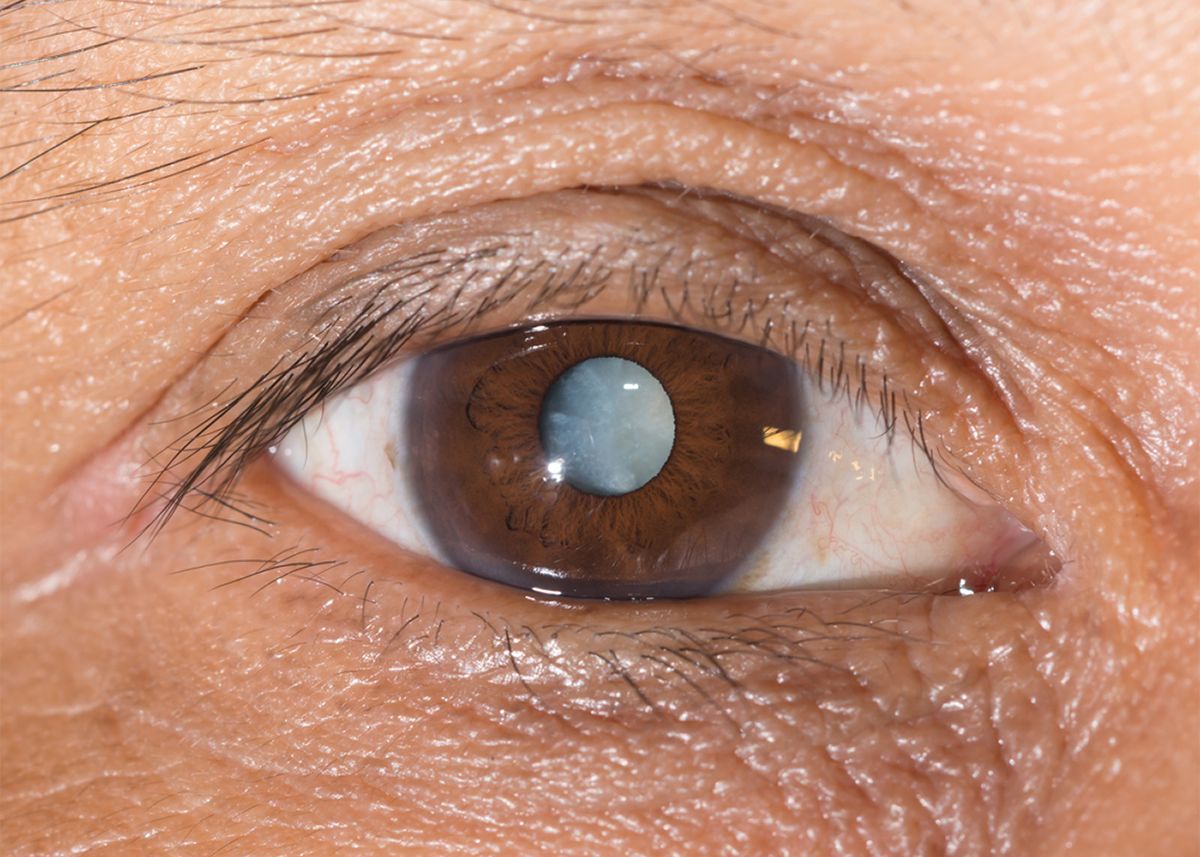The image is an extreme close-up photograph of a person's right eye, likely belonging to an older Caucasian male. The eye's iris is a deep brown color, while the pupil is an unusual blue-green hue, resembling a miniature planet like Neptune or Uranus, making the eye appear eerie and otherworldly. The white of the eye, or sclera, shows visible red blood vessels, adding to the detailed texture of the image. Surrounding the eye, the skin looks slightly wrinkled and moist, with every pore clearly visible. A portion of the right-side nostril and sparse strands of black eyebrow hair are also noticeable, emphasizing the close-up nature of this photograph.